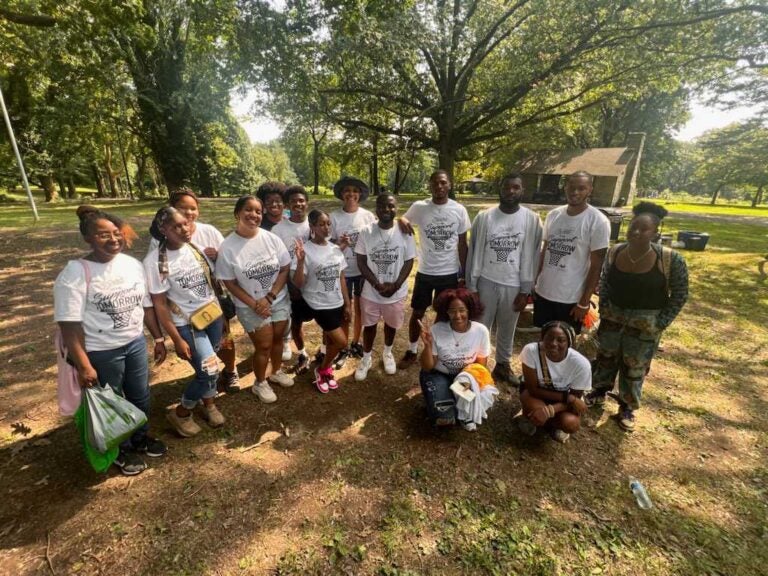The image captures a vibrant group of predominantly African-American young men and women standing together in a lush, green park. They are all wearing white t-shirts emblazoned with the slogan "Support Tomorrow," accompanied by a basketball net graphic. The group appears joyful and united, with most of them smiling warmly at the camera. Among them, a girl on the right stands out in a black tank top, a shawl, and patterned pants. The background reveals a verdant array of trees in full bloom and a small park building with benches, suggesting a communal and volunteering spirit. The ground beneath them is a mix of brown and gray dirt, reflecting the natural setting of the forest park where they seem to be participating in a camp or group activity. Everyone looks engaged and happy, potentially working together for a shared cause.